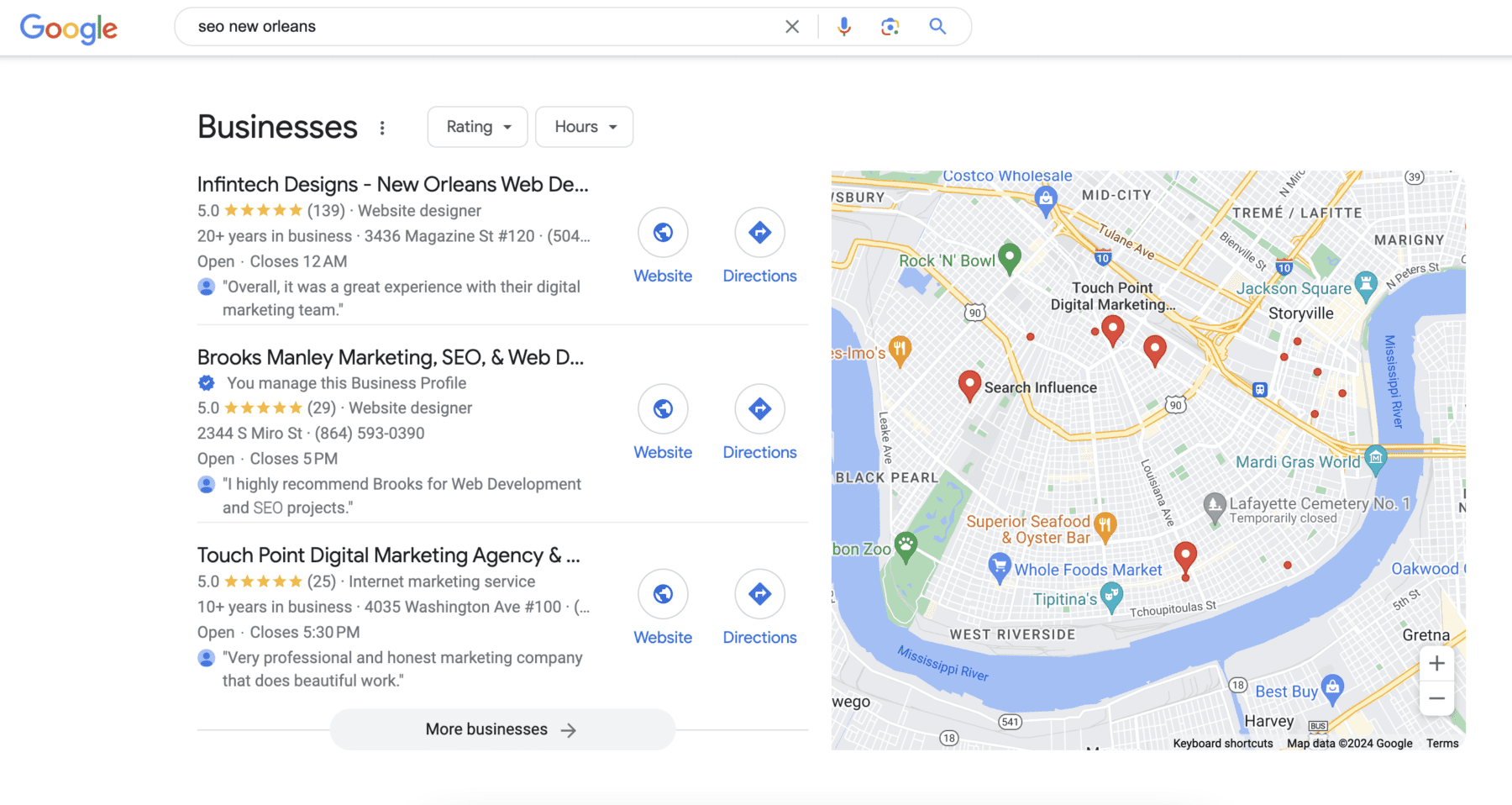This image shows a Google search result for "SEO New Orleans." On the left side, business listings are displayed, while a map with pinned locations appears on the right.

1. **Infotech Designs**:
   - **Category**: Web Designer
   - **Rating**: 5 stars (139 reviews)
   - **Location**: 3436 Magazine Street, Suite 120
   - **Years in Business**: 20+
   - **Hours**: Closes at 12 a.m.
   - **Review Highlight**: Overall great experience with their digital marketing team.

2. **Book Smart Manly Marketing SEO**:
   - **Category**: Website Designer
   - **Rating**: 5 stars (29 reviews)
   - **Location**: 2344 S Miro Street
   - **Phone**: 864-593-0390
   - **Hours**: Closes at 5 p.m.
   - **Review Highlight**: Highly recommended for web development and SEO products.

3. **Touchpoint Digital Marketing**:
   - **Category**: Internet Marketing Services
   - **Rating**: 5.0 stars (25 reviews)
   - **Years in Business**: 10+
   - **Location**: 4035 Washington Avenue, Suite 100
   - **Hours**: Closes at 5:30 p.m.
   - **Review Highlight**: Very professional and honest marketing company that does beautiful work.

Each business listing includes links to their respective websites and directions. The map on the right side is marked with pins indicating the locations of these businesses.